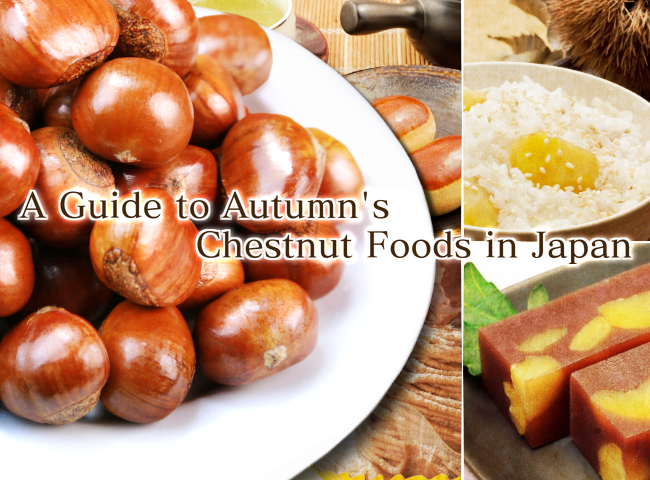The image, titled "A Guide to Autumn's Chestnut Foods in Japan," is composed of three distinct sections, each depicting various chestnut dishes. Dominating the left two-thirds of the composition is a large round white plate, possibly with a black rim, filled with whole, shelled chestnuts arranged in a heap, highlighting their rich golden-brown sheen. Against a backdrop that includes a table setting with a dish, a cup of tea, and a rolling pin or bamboo screen, this central plate suggests a warm, inviting culinary experience.

In the upper right section, a smaller image showcases a cream-colored bowl filled with white rice, possibly garnished with thinly sliced cooked chestnuts and a sprinkle of what might be panko or untoasted sesame seeds, suggesting a savory dish.

Below it, the lower right section presents a pair of brown gelatinous bars embedded with chunks of chestnut, resembling a sweet confectionery. The bars rest on a gray plate adorned with a tiny piece of green herb, enhancing their visual appeal. Together, these images collectively illustrate the diverse culinary uses of chestnuts in Japanese autumn cuisine.